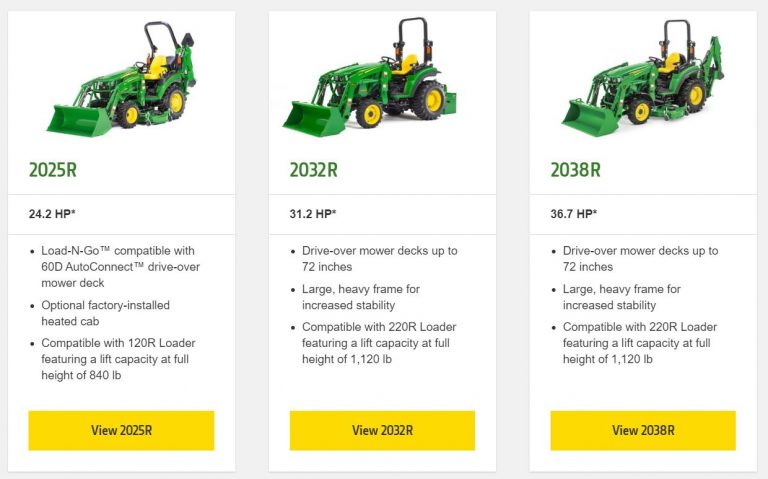The image showcases three models of John Deere drive-over mowers, each prominently displayed with specific technical details and features. The mowers are arranged in a row, all sharing the classic John Deere color scheme of green bodies, yellow seats, and yellow wheels.

The first model, labeled as the 2025R, boasts a 24.2 HP engine. It is "Load-N-Go" compatible with a 60D AutoConnect drive-over mower deck and offers an optional factory-installed heated cab. This model can work with the 120R loader, providing a lift capacity of 840 pounds at full height.

The middle model, the 2032R, features a 31.2 HP engine and supports drive-over mower decks up to 72 inches in width. It is built on a larger, heavier frame that enhances stability. This mower is compatible with the 220R loader, which has a lift capacity of 1,120 pounds at full height.

The final model, labeled 2038R, is equipped with a 36.7 HP engine and also accommodates drive-over mower decks up to 72 inches. Like the 2032R, it has a large, heavy frame for increased stability and is compatible with the 220R loader, featuring a lift capacity of 1,120 pounds at full height.

Each mower has a yellow button below it for users to view more details.